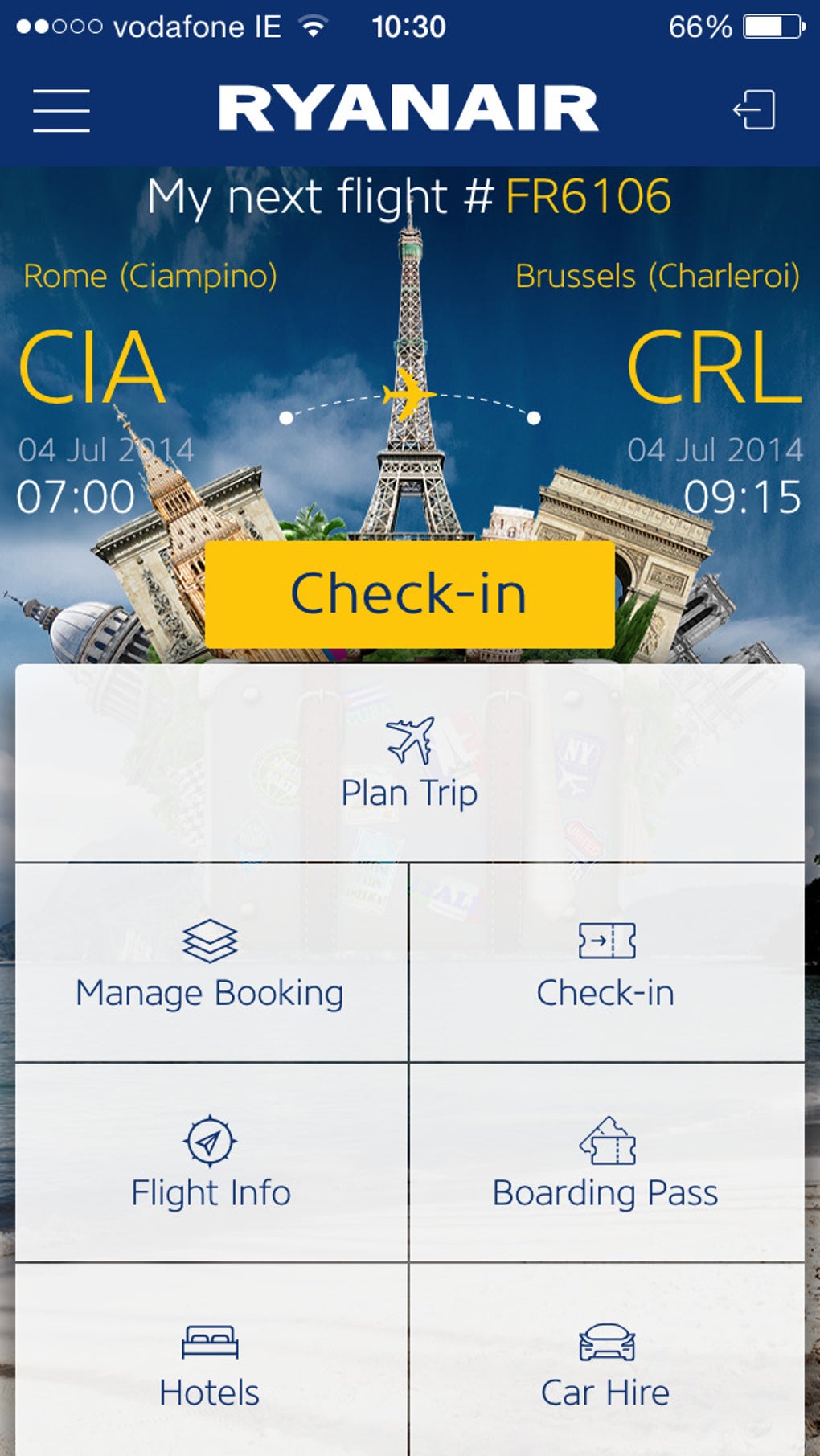The image shows a smartphone screen displaying a travel itinerary on what seems to be a travel or airline app. 

At the top of the screen, the status bar indicates the carrier as Vodafone IE with 2 dots of signal strength, a WiFi icon showing full bars, and the time as 10:30. The battery icon shows a 66% charge.

Below the status bar, the airline Ryanair is mentioned prominently. The main part of the screen centers around the details of an upcoming flight:

- **Flight Number:** FR6106
- **From:** Rome Ciampino (CIA)
- **To:** Brussels Charleroi (CRL)
- **Date:** 04 July 2014
- **Departure Time:** 07:00
- **Arrival Time:** 09:15

An icon resembling a tower, potentially symbolizing Paris, is also visible, suggesting additional travel context or information.

There is a yellow rectangle with the text "Check In." A white rectangle in the center holds the text "Planned Trip." 

Additional options are listed:

- To the left: "Manage Booking"
- To the right: "Check In"
- At the bottom: "Flight Info," "Boarding Pass," "Hotels," and "Car Hire" divided by separator lines.

The overall layout appears to be a travel app's interface on a smartphone, presumably detailing the user's next scheduled flight.